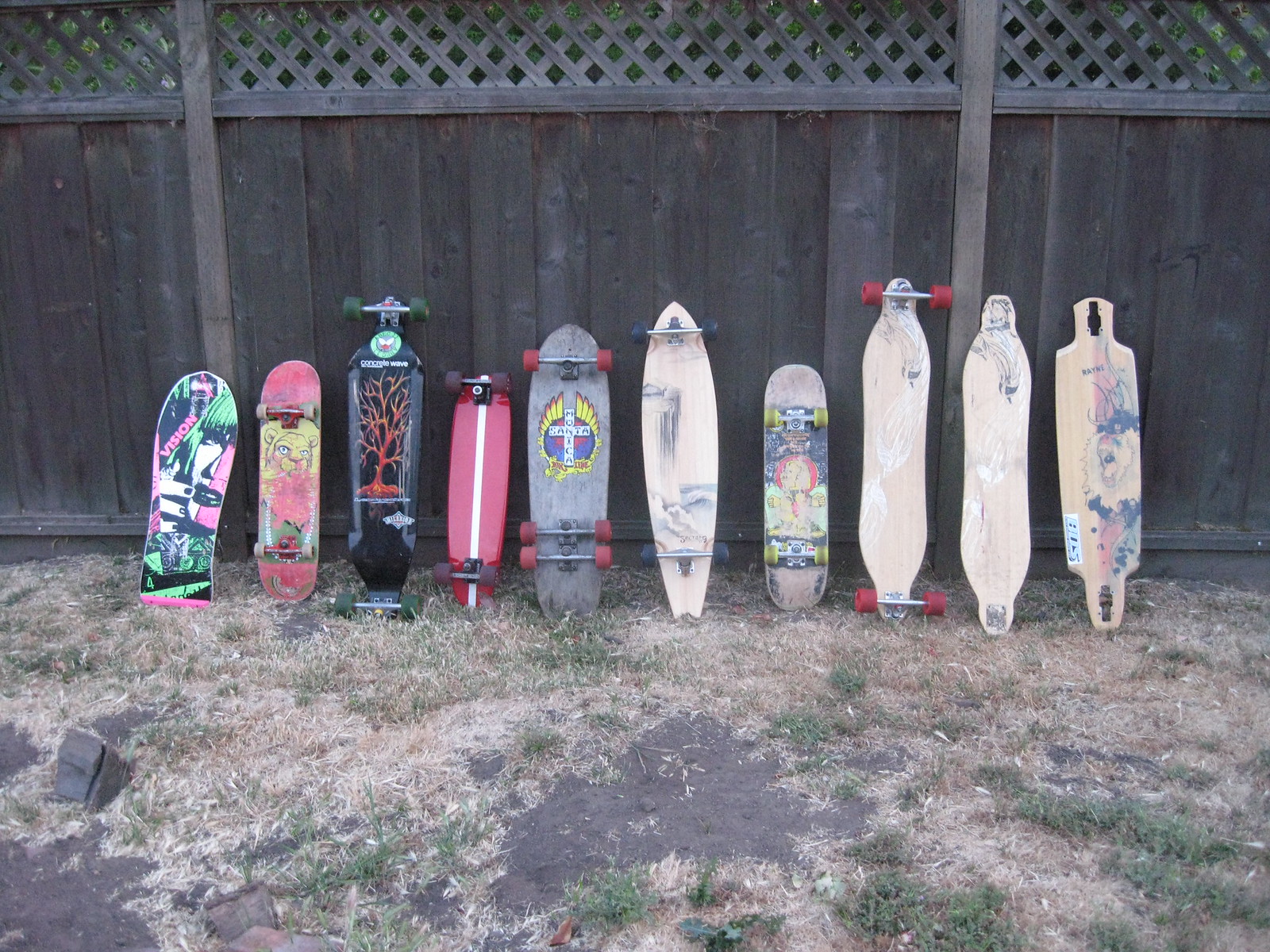This color photograph captures a weathered wooden privacy fence in a backyard. The fence features a decorative lattice design at the top, suggesting a domestic setting. Leaning against the fence are ten vertical skateboards of varying sizes, shapes, and designs. The skateboards are adorned with an array of vibrant decals, graphic images, and graffiti-style art, including intricate designs with red and pink hues, a yellowish cartoon figure, a black board with red spidery veins, and a pink board with a white stripe. Some of the skateboards sport red, green, or yellow wheels, while others are wheel-less. The yard itself is in poor condition, with dead patches of grass and sparse greenery, adding to the overall rustic and lived-in feel of the scene.